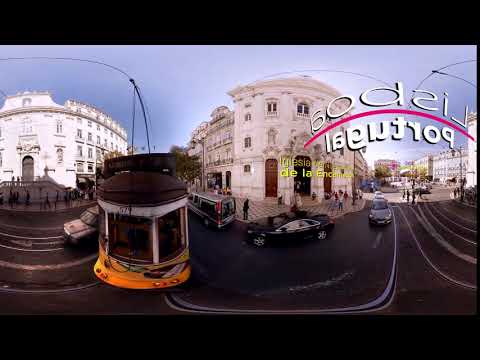The image appears to be taken from a high vantage point, possibly from a surveillance camera. It captures a city street scene with a bustling atmosphere. In the foreground, there's a white building on the left with brown trim and a brown door, accented by white stairs. This building has several windows and red doors on its sides. People are visible on the brownish-tan sidewalk, dressed mostly in dark clothing, while some stand out in white shirts, blue pants, and red shirts. The street below features a white left-facing arrow and lines indicating traffic direction. A trolley with the number 579 in black on a white background, colored in brown, white, and yellow, runs through the center of the image. Near the trolley, a black and white van, a black car, and a gray car are present. In the background, there are additional buildings mostly white with brown doors, and some have green trees around them. The sky is blue with white clouds, giving a bright outdoor ambiance. Text on the image includes "LISBOHORCHICLE" in white letters with a curved pink line between, and "DELA ENCANTA..." in yellow letters. The scene exudes the hustle and bustle of a city area, with elements such as a possibly foreign word "Portage" indicating a transitory or transport-related location.